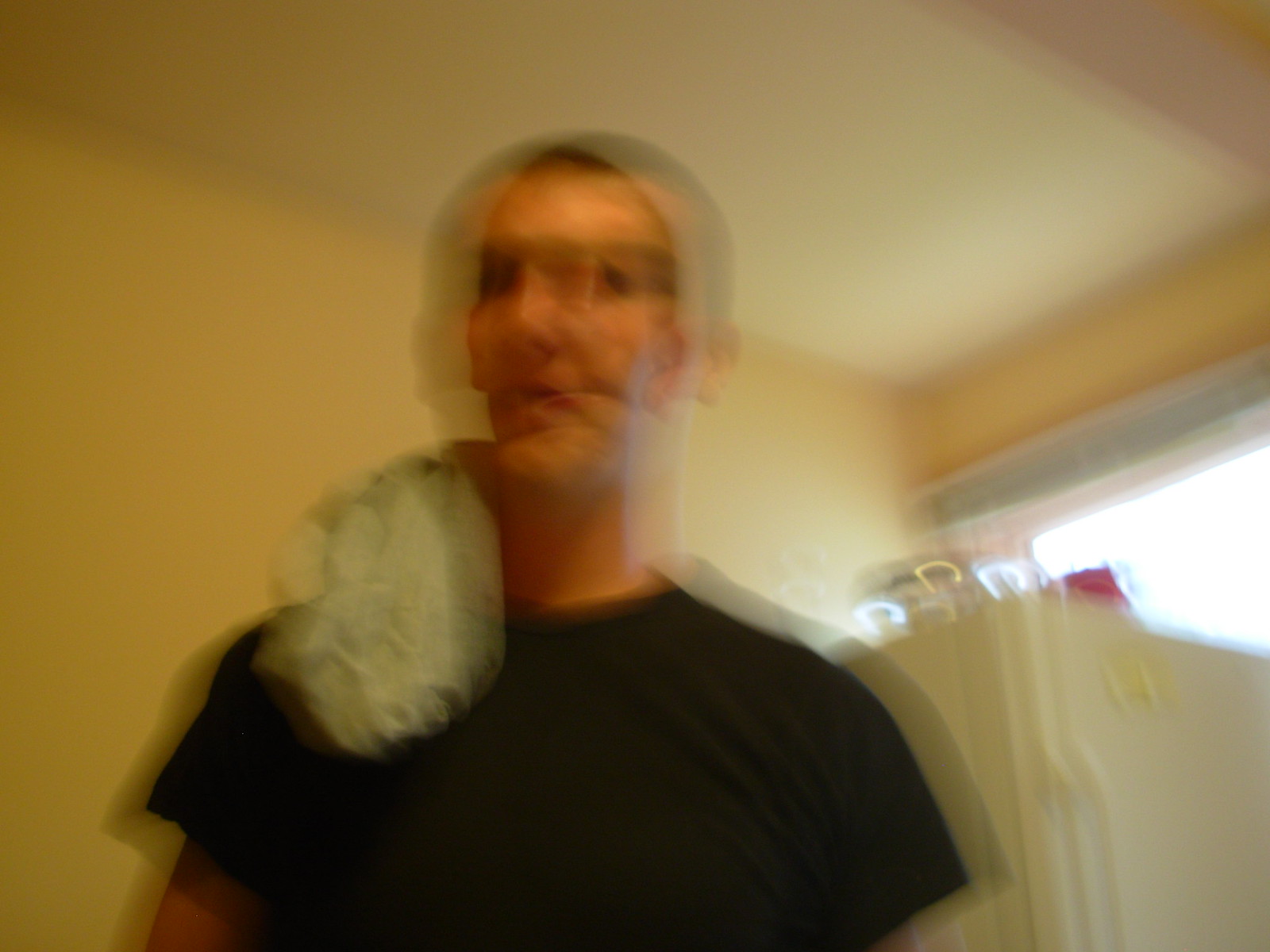In this exceptionally blurry photograph, a male figure with an almost shaved head is depicted wearing a black t-shirt. Perched on his shoulder is an indistinguishable object, possibly a towel, pet, or creature, rendered unclear due to the photo's lack of focus. The scene appears to be indoors, identifiable by the yellow wall and white ceiling in the background. Additionally, a white appliance, likely a refrigerator or freezer, is visible to the left of the subject. Notably, the image is devoid of any text, emphasizing its enigmatic and unfocused nature.